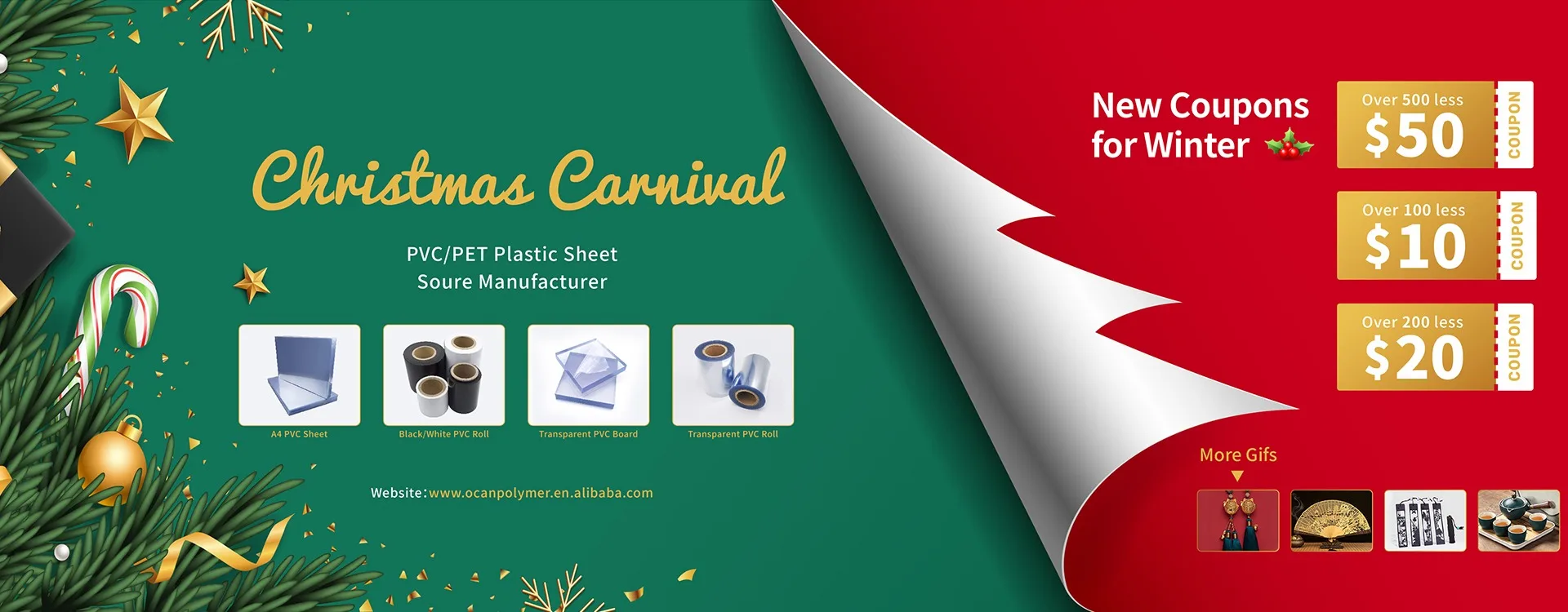This festive advertisement, designed for the Christmas season, showcases a variety of PVC products in a visually appealing format. On the left side, there's a prominent title that reads "Christmas Carnival," followed by text advertising "PVC/PET Plastic Sheet" and "Source Manufacturer." Below this, there are four white squares, each featuring an image and description of different products: "Add PVC Sheet," "Black/White PVC Roll," "Transparent PVC Board," and "Transparent PVC Roll." Additionally, the company's website, www.ocanpolymer.en.alibaba.com, is displayed.

The entire background radiates holiday spirit, adorned with Christmas-themed decorations such as candy canes, a partial view of a tree, stars, and golden embellishments. On the right side of the ad, the image creatively peels back to reveal a white Christmas tree. This section highlights new winter coupons with denominations of $50, $10, and $20, along with an enticing "More Gifts" caption and several gift images at the bottom. The festive elements and product highlights are seamlessly integrated, making it a captivating holiday advertisement.